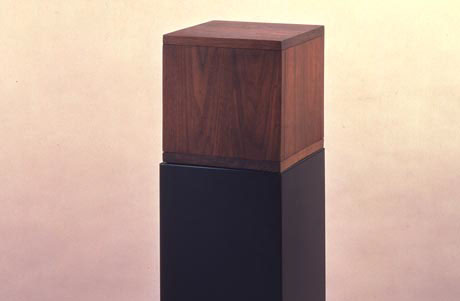In this artwork, the background gradually transitions from a very pale yellow at the top to a soft pink and finally to a subtle purplish hue at the bottom. At the center, there are two cubes, arranged such that the entire composition appears horizontal and rectangular but relatively small. The top cube is a textured wooden box with visible wood grain, rendered in a tan-brown color. This wooden cube is slightly shorter and positioned a bit to the right, showing its three-dimensional form at an angle. Below it, there's a solid black cube that extends downwards, separate from the wooden one, as indicated by a slight misalignment at the edges. The light source behind the cubes creates a reflective effect on a glass-like surface, which results in the appearance of a darker, black reflection of the wooden box. The background around the cubes appears hazy, shifting from a soft peach to grayish tones, adding to the ethereal quality of the image. The scene’s lighting highlights the contrast between the warm tones of the wooden cube and the starkness of the black one, making the detailed intersections and reflections visually compelling.